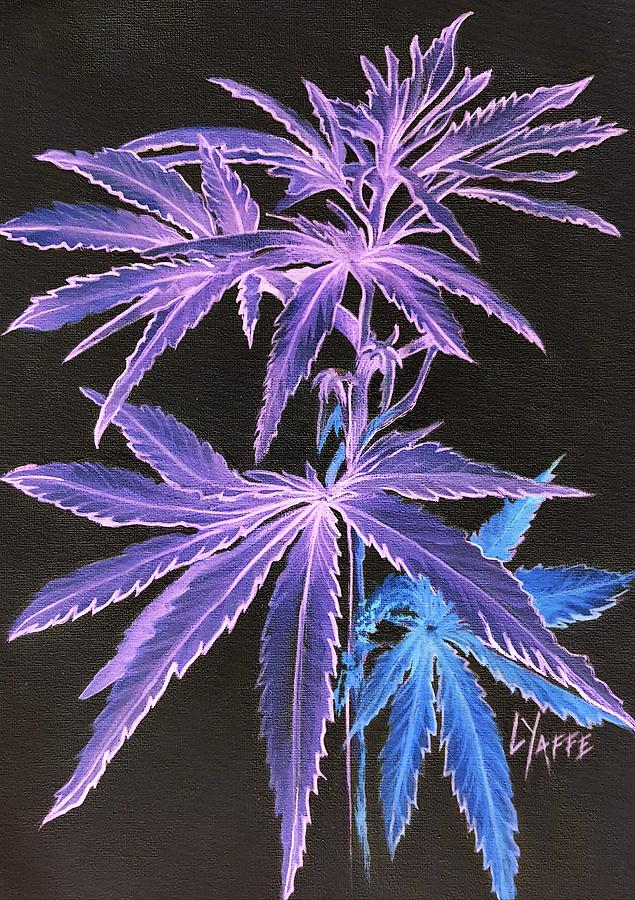The image is a detailed illustration resembling a marijuana plant, set against a black background. The plant is depicted with neon-colored hues, featuring primarily purple leaves with a noticeable blue auxiliary leaf. The leaves, numbering around seven, fan out in a starburst pattern typical of a marijuana leaf, with the larger leaves at the bottom and smaller ones towards the top, culminating in what appears to be a small bud. The purple leaves exhibit a gradient towards their center, transitioning to lighter pinkish or almost white hues. The plant's stalk is thick at the base and tapers towards the top. The rectangular canvas, marked by a signature in the bottom right corner reading "L-Y-A-F-F-E," measures approximately in a 2:3 height-to-width ratio, indicating the work of the artist.